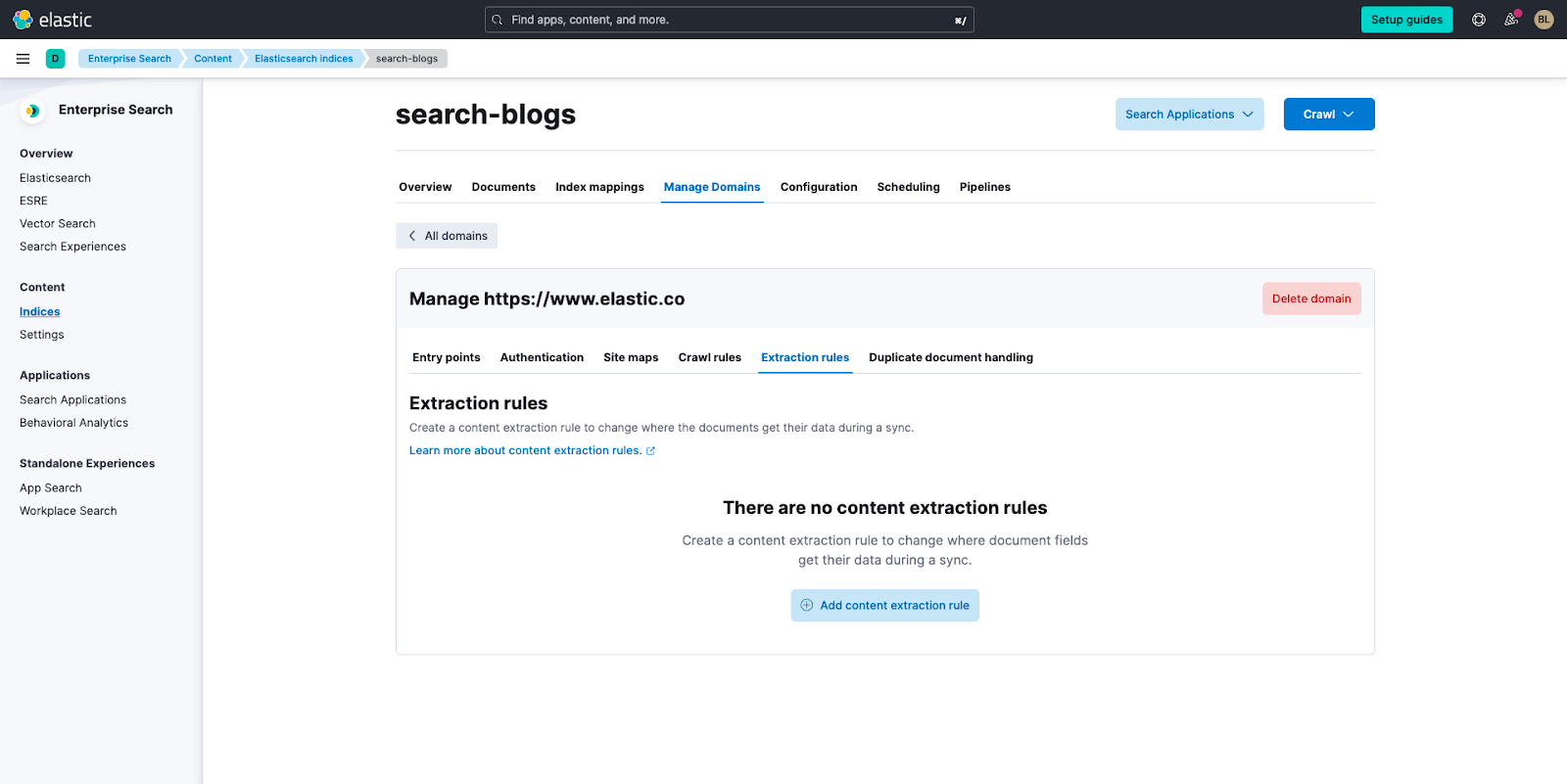This image depicts a screenshot of a search blog website named "Elastic." The website's name, "elastic," is displayed in the upper left corner in lowercase white font. The logo, situated next to the name, is a collection of colorful, rainbow-like bubbles. A black navigation bar spans the top of the page, featuring a centrally positioned search bar.

In the upper right corner of this navigation bar, several options are visible: "setup guides" and three additional buttons. The main page itself is titled "Search Blogs" and provides options to manage the website, specifically at the URL https://www.elastic.co. It notes that there are no content extraction rules set, offering the user the options to either delete the domain or add new content extraction rules.

The overall design of the website is clean and straightforward, characterized by a predominantly white background.